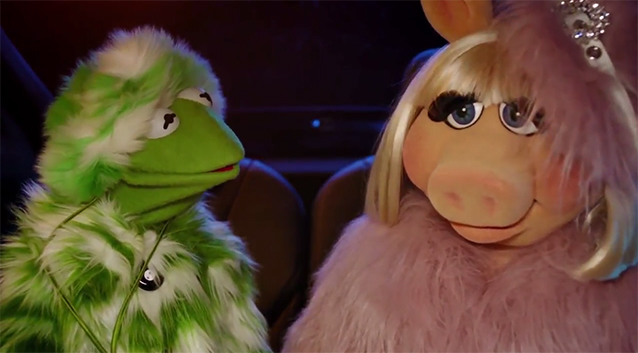The image features two iconic characters, Kermit the Frog and Miss Piggy. Kermit is positioned on the left, dressed in a distinctive green and beige fur outfit that resembles a hat and coat. His prominent features include a green nose, white eyes with black slit pupils, and a red tongue. There's something black with a white center on his chest, likely a button. Kermit's gaze is directed towards Miss Piggy, who sits on the right.

Miss Piggy is adorned in a pink fur hat and a matching pink furry jacket. Her shoulder-length blonde hair complements her look, and she sports large false eyelashes and pink cheeks. Miss Piggy's eyes are focused straight ahead. Both characters are seated in what appears to be a dimly lit setting, possibly the back of a car or a movie theater, suggested by the dark background and the nature of their chairs. The scene captures a moment of quiet interaction between the two, with Kermit observing Miss Piggy and her poised demeanor.